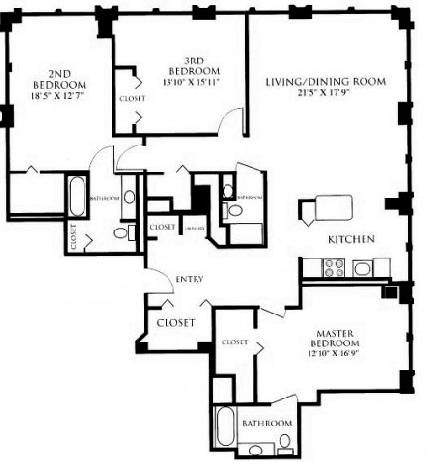This detailed floor plan features a well-thought-out layout starting from the entryway, where you'll find two closets, one on the right and another on the opposite side. Proceeding forward and turning right leads you to the master bedroom, which includes a walk-in closet and an en-suite bathroom. 

Continuing straight from the entryway, you enter the kitchen, which boasts an island at its center. Adjacent to the kitchen on the left, you'll discover a spacious living room and dining area. 

Parallel to the entryway, there is another hallway located on the other side of the closets, kitchen counter, and a wall. Following this secondary hallway, the first door on the left opens into a powder room, succeeded by an additional closet. On the right side of this hallway lies the third bedroom, which has its own closet but does not feature an en-suite bathroom. 

Moving further down the hall, you reach the second bedroom, complete with its own shower, toilet, and a walk-in closet. The master bathroom is also equipped with a walk-in closet. The architectural design ensures ample storage and functionality throughout the home.